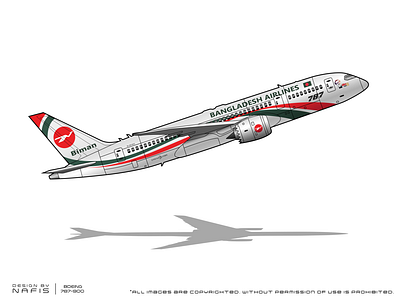This is a detailed computer-generated illustration of a passenger aeroplane taking off, angled to emphasize its ascent. The aircraft, a Boeing 787, belongs to Bangladesh Airlines as indicated by the gray text "Bangladesh Airlines" near the front of the plane. The aeroplane's body is white with red and green wavy lines that also feature on the rudder. Prominently displayed near the nose of the aircraft is the number 787. The plane's tail features a striking red circle enclosing a white bird image, below which is the name "Biman" in gray. The illustration has a thick black outline that gives it a slightly cartoony appearance, and it’s set against a flat white background with a subtle gray shadow below depicting the plane’s ground reflection. The landing gear is retracted, further emphasizing that the plane is in mid-takeoff. Additionally, small text in the lower left-hand corner states "designed by NAFIS," and clarifies that all images are copyrighted, prohibiting use without permission.